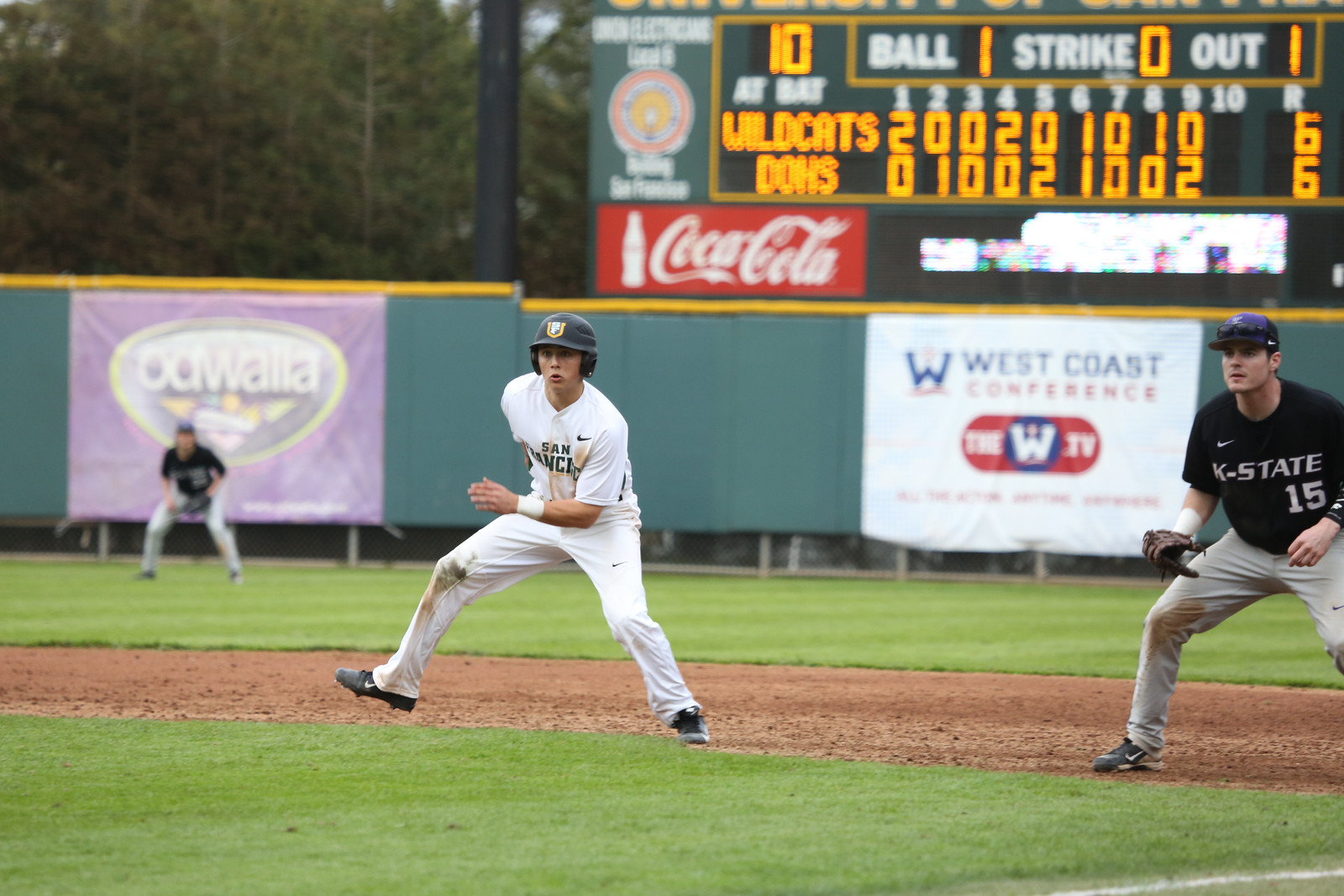The image captures a dynamic moment during a daytime baseball game at an outdoor field. Central to the photo is a young Caucasian player, possibly in his late teens or early twenties, dressed in a white uniform and helmet. He appears to be preparing to run, with one foot raised. To the right, another player in a dark jersey marked "K-State 15" and white pants stands with a catcher's mitt ready for action. In the backdrop, a third player in a dark shirt and white pants is seen bending over. The background features a tall green wall adorned with advertisements, including prominent ones for Coca-Cola and West Coast Conference, alongside a scoreboard displaying a tied score of 6-6. The scoreboard also shows the team names "Wildcats" and "Dons," highlighting the competitive tension of the moment.